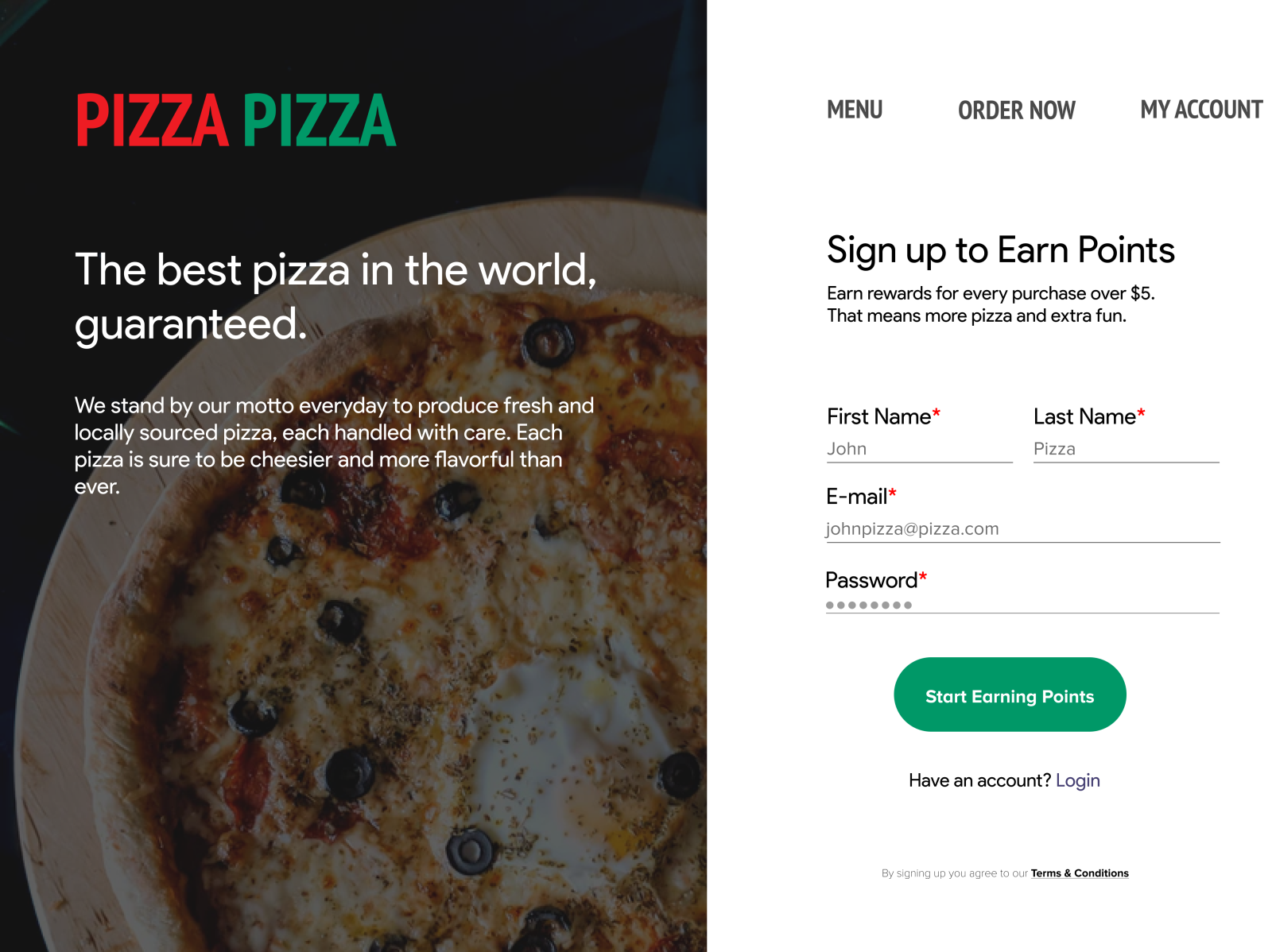**Descriptive Caption:**

A screenshot from an unidentified pizza restaurant website. On the left side, there is a mouth-watering photograph of a pizza topped with melted cheese, ripe tomatoes, and sliced black olives. The header features the text "Pizza Pizza," with "Pizza" in red letters and the second "Pizza" in green letters. Beneath this header, a slogan reads: "The best pizza in the world guaranteed. We stand by our motto every day to produce fresh and locally sourced pizza, each handled with care. Each pizza is sure to be cheesier and more flavorful than ever."

On the right side of the screenshot, several navigational and promotional options are displayed, including "Menu," "Order Now," "My Account," and "Sign up to earn points." A promotional note encourages customers to "earn rewards for every purchase over $5," promising "more pizza and extra fun." The sign-up form requests a first name (John), last name (Pizza), email (JohnPizza), with the password being redacted and a prompt to start earning points. Below the form, there is an option to log in for those who already have an account, with a reminder that signing up indicates agreement to the website's terms and conditions. 

The image contains no people, animals, plants, flowers, trees, automobiles, motorcycles, or airplanes.